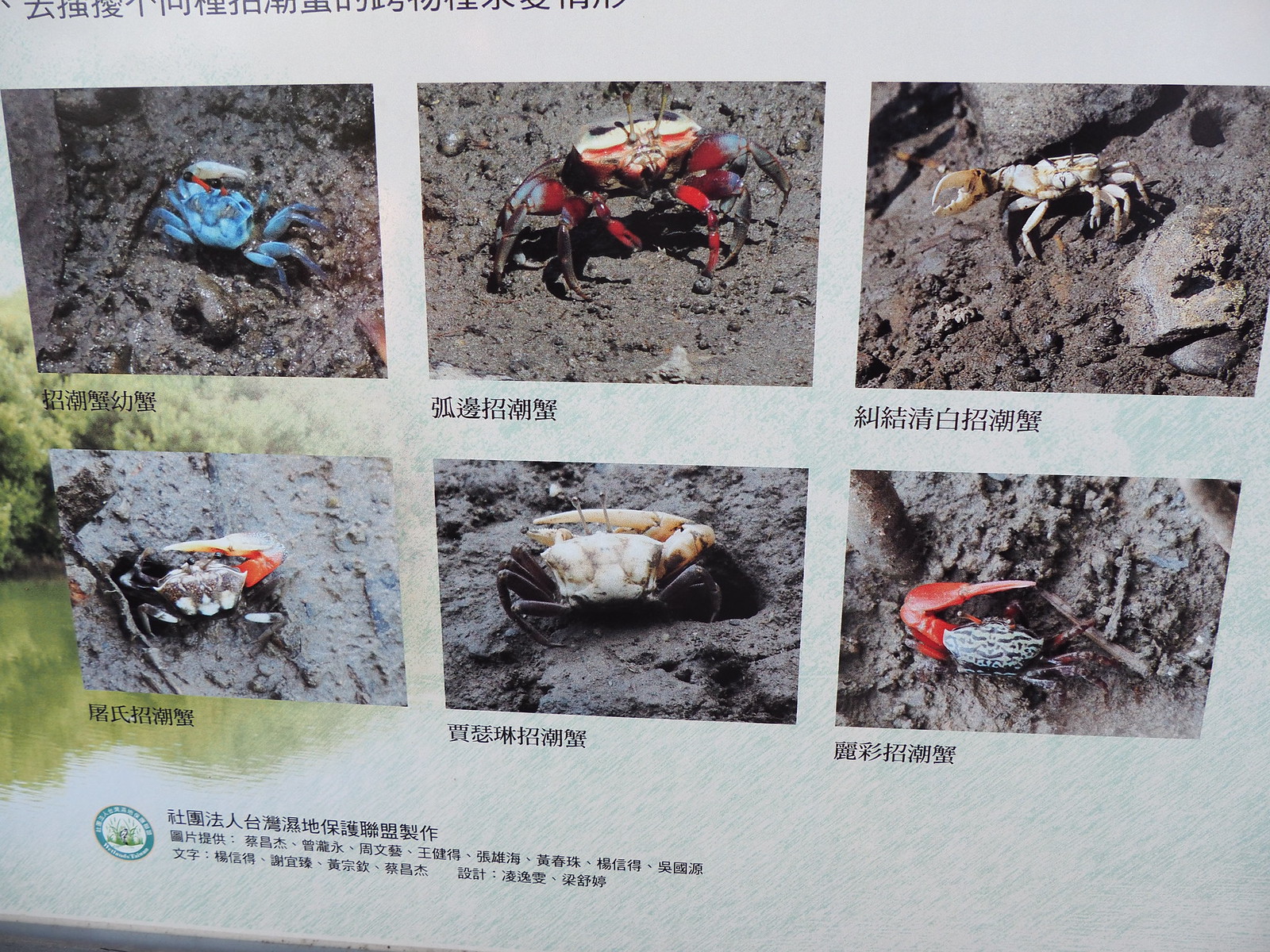The image shows a printed piece of light orchid-colored paper featuring six detailed photos of different crabs, each accompanied by non-English text, possibly Chinese, at the top, bottom, and underneath each image. Starting from the top left is a striking blue crab. Next is a slightly larger crab with a mix of cream, red, and a hint of blue. The third crab in the top row is predominantly cream-colored. On the bottom row, the first crab on the left is primarily gray with a distinct red pincher. The fifth crab displays a white body and pincher, contrasted by its black legs. The final crab has a distinctive striped black and white body, complemented by brown legs and a red pincher. The background includes green grass and a large tree on one side, juxtaposed against muddy beaches.